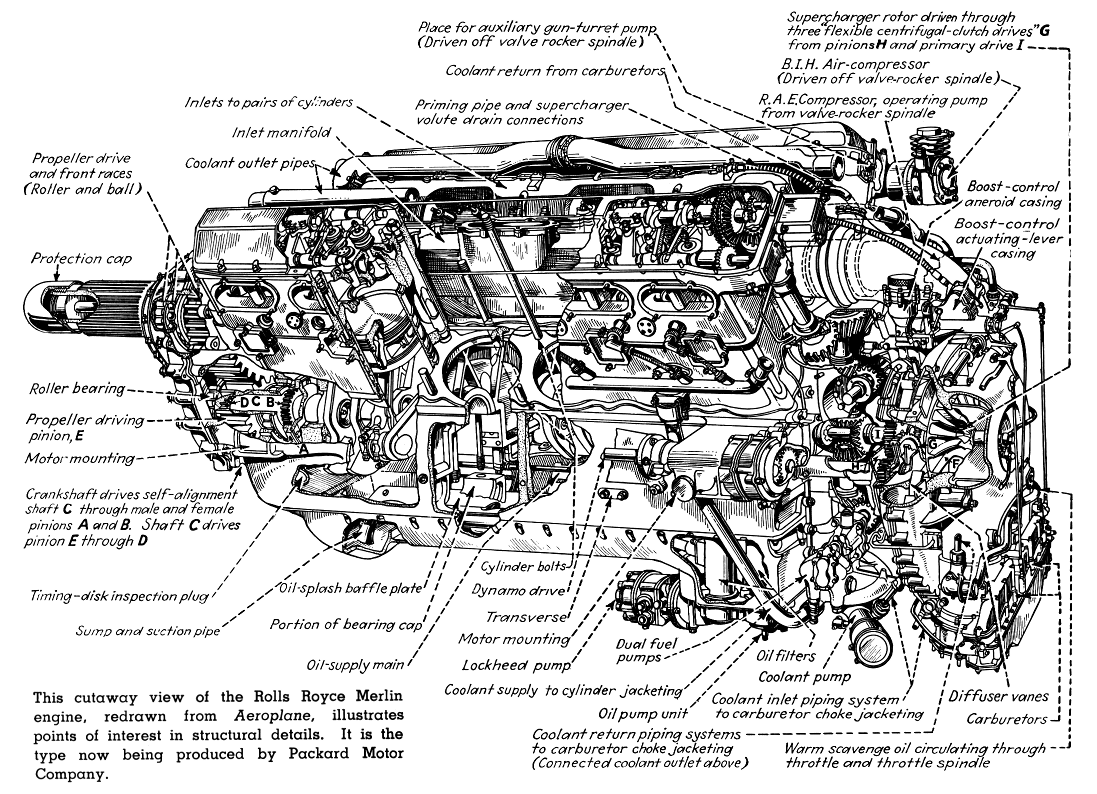This highly detailed black and white schematic illustrates the intricate components of the Rolls-Royce Merlin engine, now produced by Packard Motor Company. Redrawn from the publication "Aeroplane," this cutaway view highlights key structural details and points of interest. Every part of the engine is meticulously labeled, with dotted lines extending from each component to its corresponding label. Prominent parts identifiable in the image include the protection cap, roller bearing, propeller driving pinion, motor mounting, crankshaft, oil splash baffle plate, bearing cup, oil supply, main oil filters, coolant pump, carburetors, and oil pump unit. The image is enriched with a variety of gears and metallic pieces, depicting an extensive and comprehensive layout of the engine. The description at the bottom left corner, written in a bold black font, provides context and emphasizes the significance of this intricate engine design.